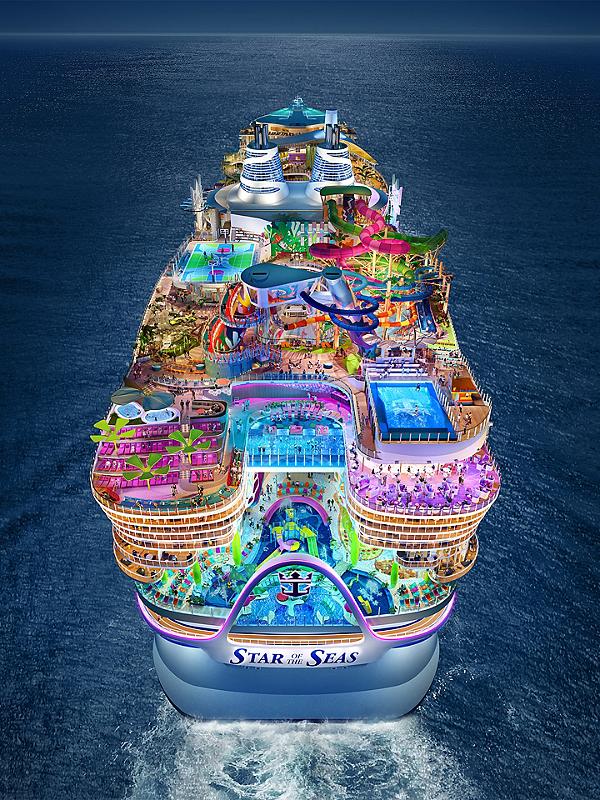The image is a computer-rendered depiction of an enormous cruise ship titled "Star of the Seas" on the open, dark blue sea at nighttime. The ship, prominently centered, is white and filled with intricate details that embellish its grandeur. It is sailing away from the viewer, evident by the wake trailing behind it. The design showcases multiple levels, teeming with activities and amenities. Neon lights in hues of pink, purple, blue, and green illuminate water slides that snake across the top deck, alongside at least one pool. The ship’s complexity is highlighted by detailed features, including an anchor symbol arched above the ship's name at the stern. Other visible elements suggest various recreational facilities like sports fields, trees and greenery, possible restaurants, discos, and theaters. The stillness of the dark sea contrasts with the vibrant and active ambiance aboard the ship, enhancing its imposing presence against the night sky.